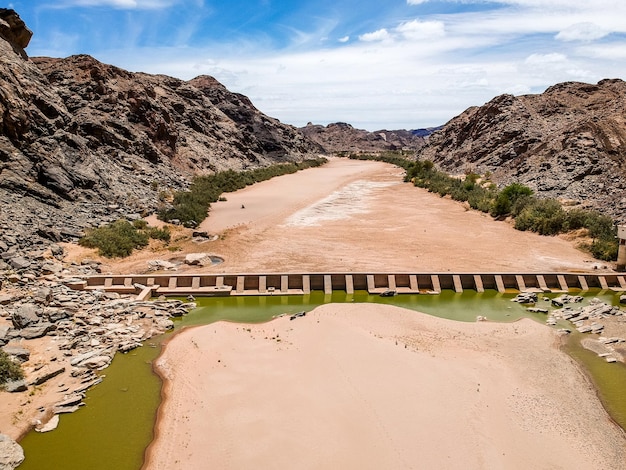The image captures an aerial view, likely taken by a drone or helicopter, of a desolate landscape dominated by an old, concrete dam that stretches horizontally across the center. This dam, now seemingly defunct, intersects a dry riverbed that's enveloped by a barren, light brown sandy desert. Below the dam, there are supporting pillars embedded into the structure. The lower region of the image features a small island of sand surrounded by sparse, greenish-grey water that pools slightly at the center and along the left and right edges. The banks of the riverbed display a medley of rocky outcrops and sand, with dark green brush sporadically dotting the terrain. In the background, rocky hills or small mountains rise up on either side, with the sky above them filled with a mixture of blue patches and swirling white and grey clouds, adding to the stark, isolated feel of the scene.